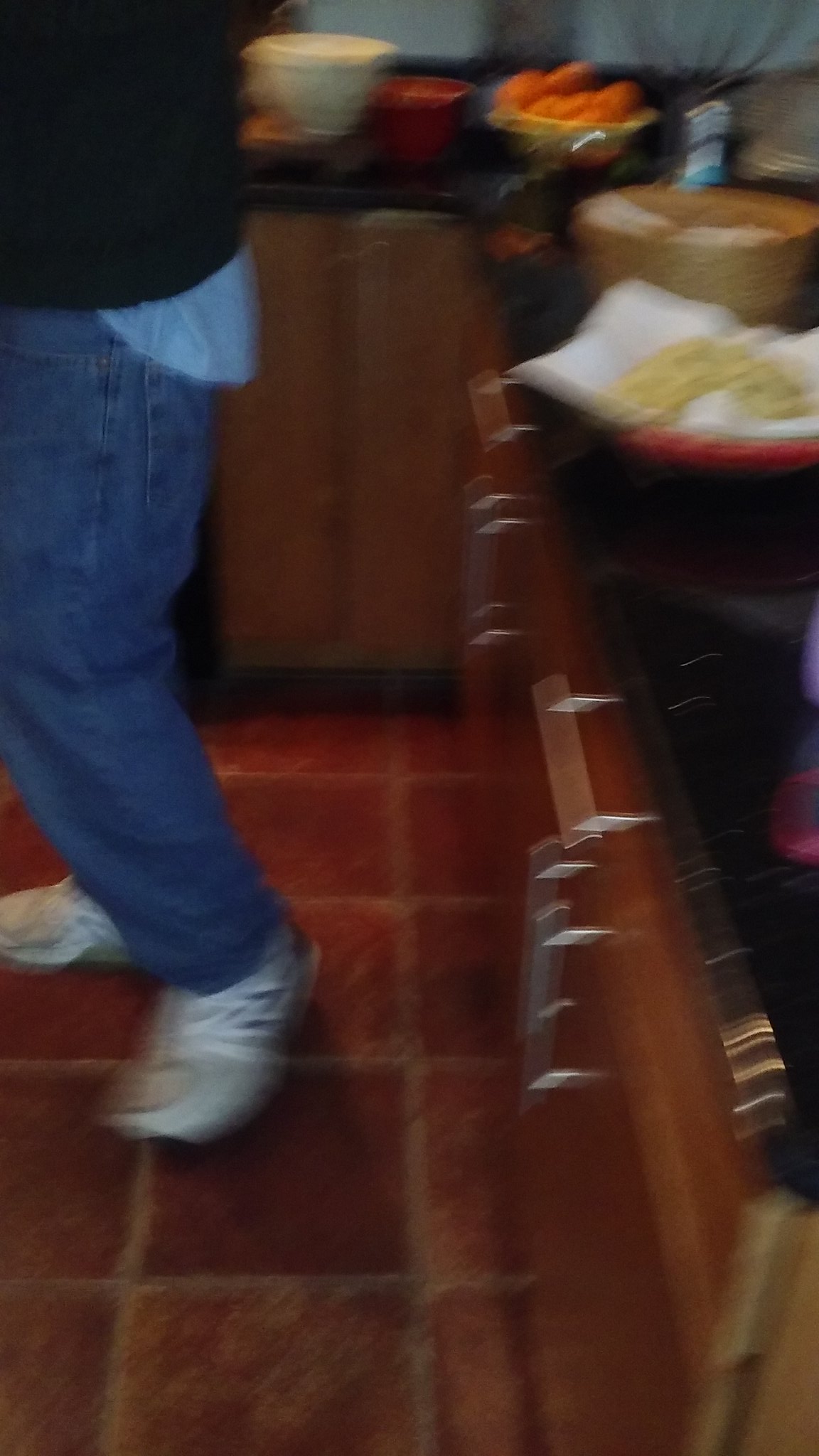An indoor color photograph portrays a dimly lit and heavily blurred kitchen scene. The image is taken looking slightly downward along a blackened kitchen countertop on the right, under which several medium brown wood cabinet doors are visible, equipped with shiny silver or stainless steel handles. The countertop itself hosts a couple of baskets containing indeterminate food items due to the photograph's poor focus. Adjacent to the countertop, a person is captured mid-step, moving away. This individual, whose gender is not discernible, is dressed in blue jeans, a darker shirt with a blue shirt tail peeking out, and white sneakers, with the left foot appearing blurred in motion. The floor beneath is a brownish-orange tile.